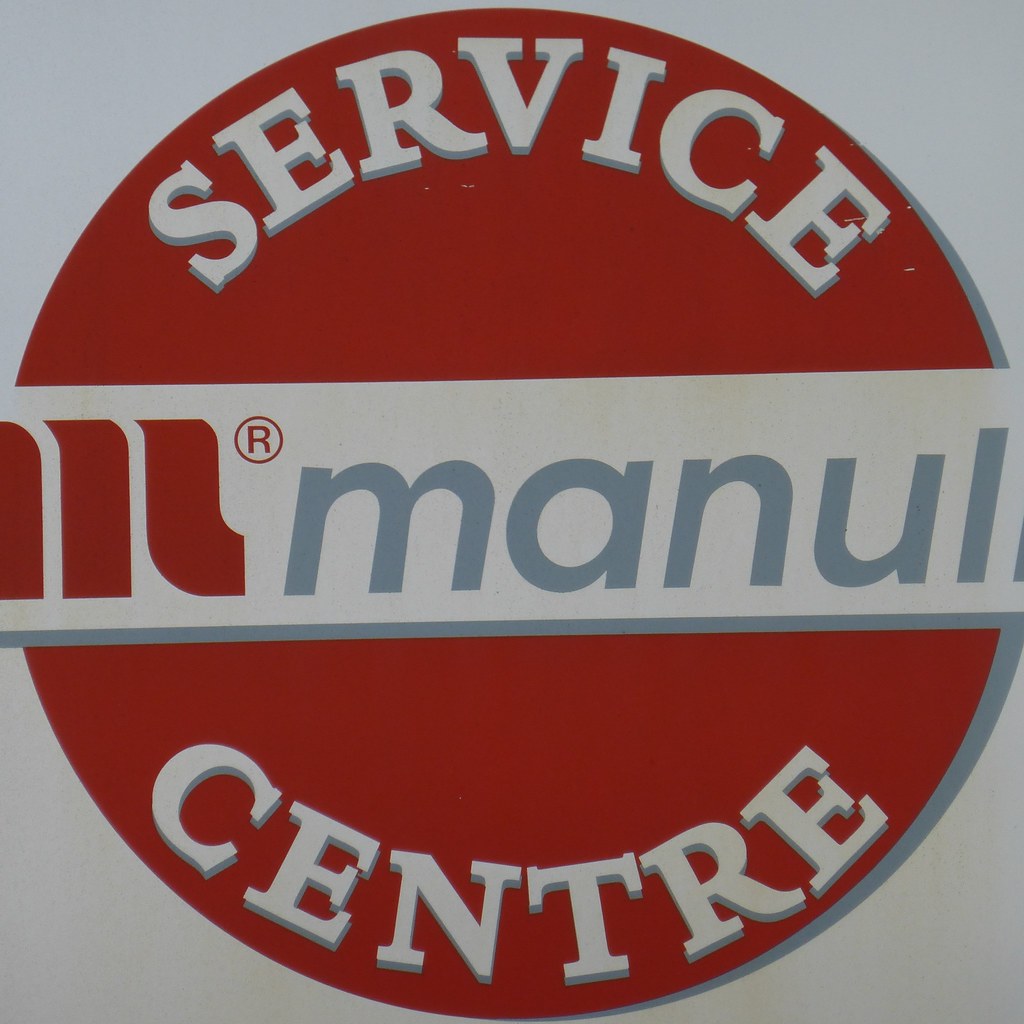The image is a vertically-oriented, close-up photograph of a business sign, set against a grayish-white background. Dominating the entire rectangular sign is a large red circle. Within this circle, the word "Service" is prominently displayed at the top in large, white uppercase letters, and the word "Center" appears at the bottom in matching font and color. Cutting across the midpoint of the red circle is a slightly off-horizontal gray band. On the left end of this gray band, partially cut off, are three small red lines resembling an ad logo, accompanied by a red registered trademark symbol (a red "R" inside a circle). Beside these elements, it reads "MANUL" in lowercase gray letters. The detailed alignment and striking color contrast make the sign highly noticeable.